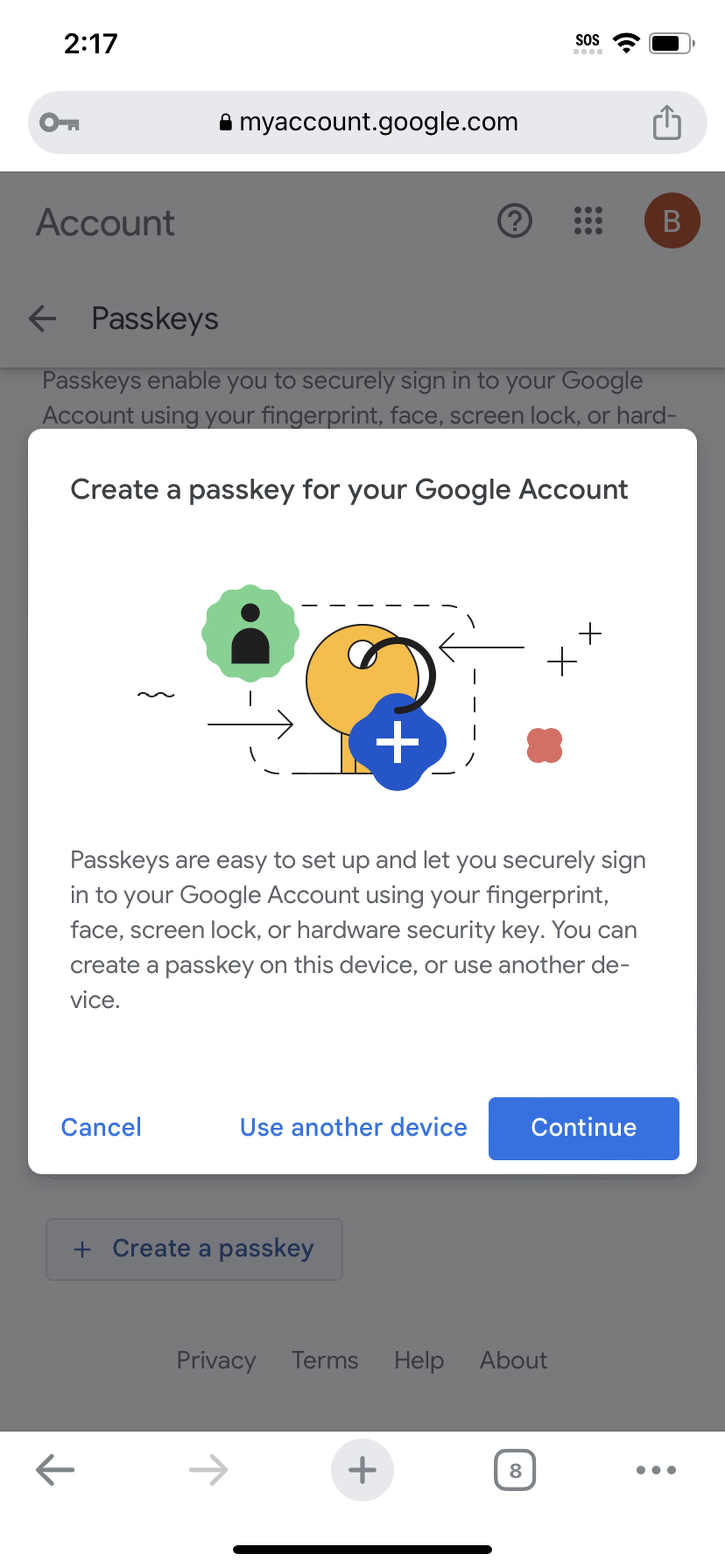The image captures a detailed screenshot of a mobile device screen displaying a Google page. 

- In the top-left corner, the time is shown as 2:17. 
- To the right of the time, the signal status indicates "SOS" mode, implying no cellular signal, accompanied by the Wi-Fi symbol, and the battery icon showing a charge between 75% to 80%.

Immediately below this bar:

- The Google page is evident with an account count visible on the top-left.
- On the top-right of the Google page, there are several icons including a "Help" button, a menu tab, and a profile avatar featuring a bee inside an orange circle.

Central to the screenshot:

- The user has engaged with a section titled "Passkeys".
- A prominent white square pop-up appears, detailing "Create a passkey for your Google account".
- This pop-up includes a visual representation of a passkey, with an icon of a user inserting into a gold key with a blue plus sign attached.

Below this illustration, descriptive information about passkeys and their role in signing in are provided. 

At the bottom of this white pop-up:

- Three buttons are visible: "Cancel" on the bottom-left, "Use Another Device" in the center, and "Continue" on the bottom-right.